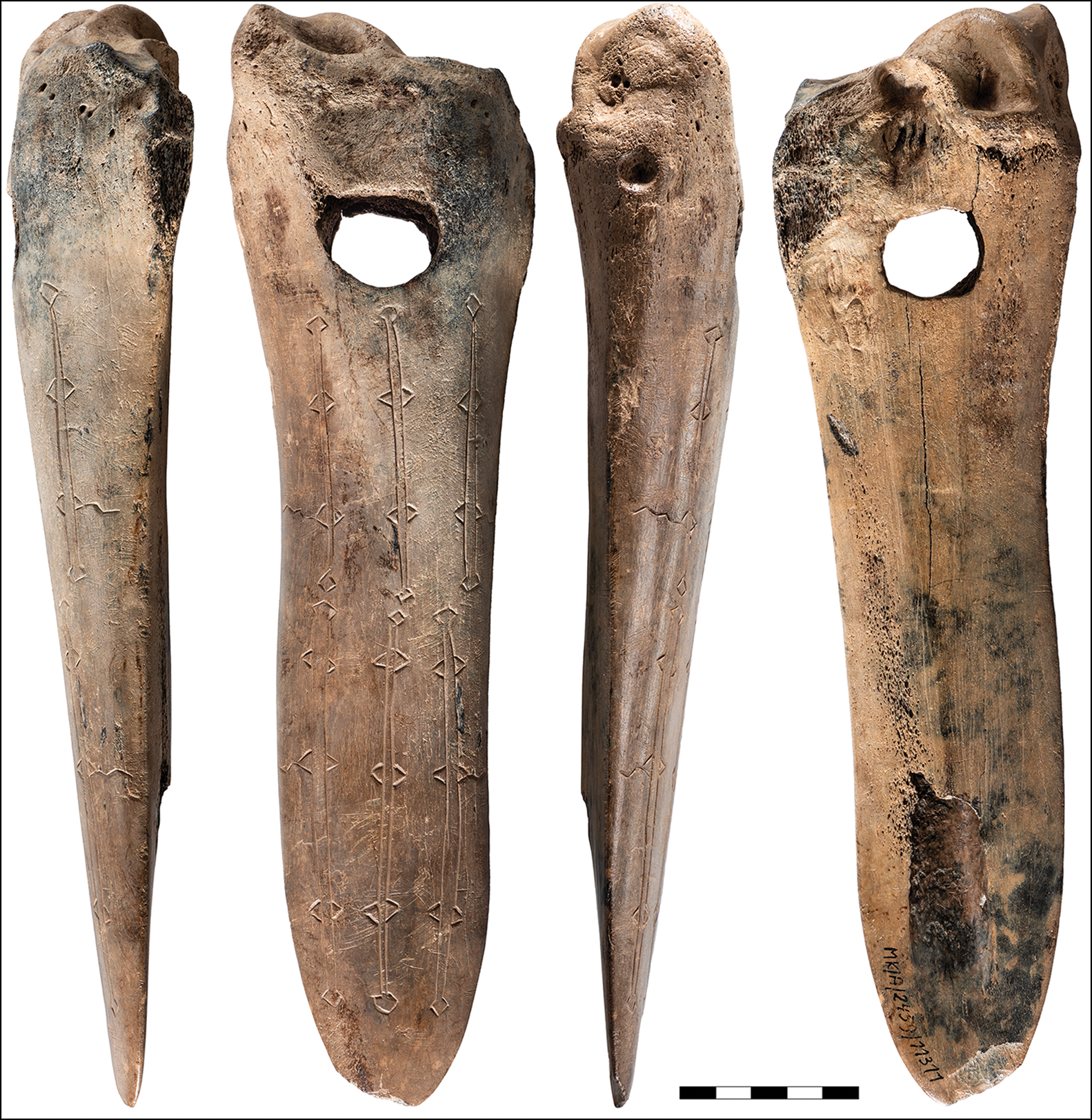The image depicts four long, thin bones that appear to be ancient artifacts, likely excavated by an archaeologist. These bones, which may be animal bones or prehistoric tools, feature intricate carvings. The carvings consist of vertically etched diamond-shaped and line patterns, positioned in rows. One side of each bone showcases these detailed designs, while the other side remains bare. Notably, two of the bones are pointed and have a single hole drilled at their top, whereas the other two bones have two holes each drilled into them. The bones are displayed against a white background, and there is a small scale beneath the bones, indicating their size. The bones are presented in different views, similar to how they might be showcased in a scientific journal or museum exhibit, suggesting meticulous documentation of these intriguing relics.